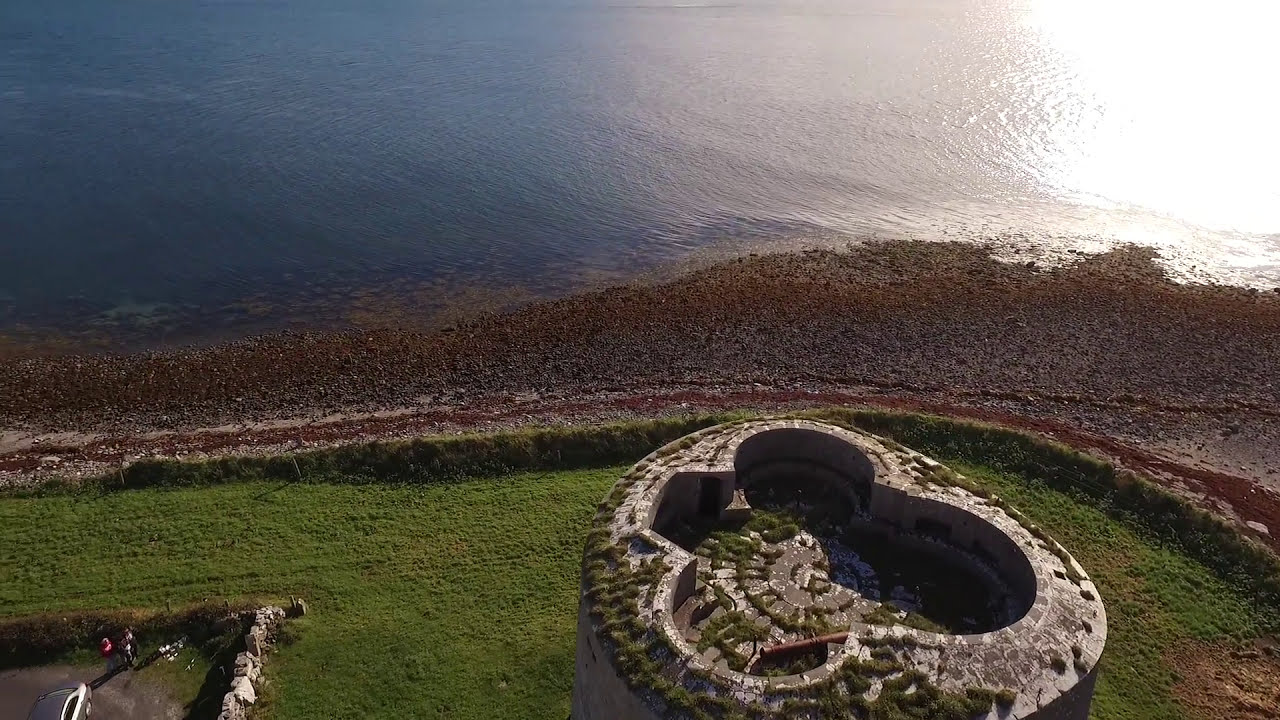This is an overhead view, taken from approximately 40 feet above, of a rural seaside area featuring a beach with a purplish hue, possibly due to scattered shells. The upper third of the image shows a body of water—perhaps an ocean or large lake—with a bright reflection of sunlight in the upper right corner. The coastline is rocky and extends horizontally across the image, curving slightly downward at the right edge.

The middle section of the image showcases a brown, rough clay-like terrain transitioning into a more grassy, green area in the foreground. The focal point is a man-made, circular stone structure with a deep cutout resembling a clover pattern. The structure appears ancient, with green moss and brown patches, indicating possible concrete and bushes.

In the lower left corner, there is a bordered-off area with rocks and a mix of grass and dirt, where two or three people are visible near a silver parked car. The main colors are blue, white, purple, tan, and green.